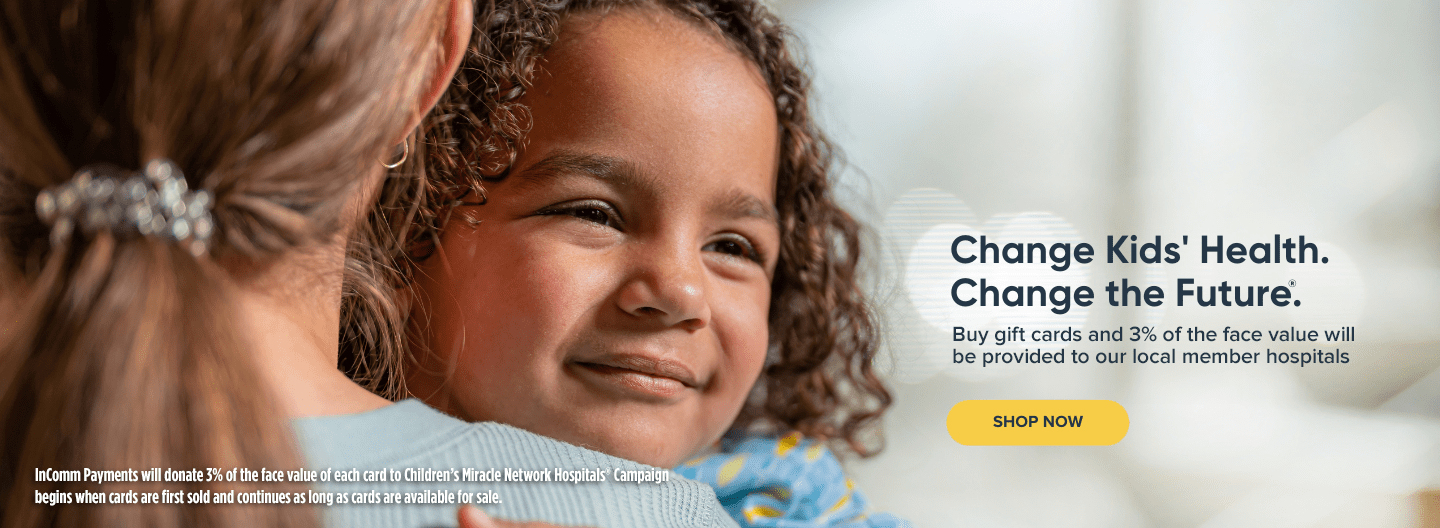The website features a heartwarming image centered on a mother and her child. The back of the mother is visible, emphasizing her sleek ponytail adorned with a sparkly, silver ponytail holder that resembles stone. She is dressed in a light blue, waffle-textured shirt. Embracing her child lovingly, the child's face is turned to the left, smiling without showing her teeth. The child has brown, curly hair and appears to be wearing light blue pajamas decorated with orange and yellow designs. 

To the right side of the image, the text "Change Kids’ Health, Change the Future" is prominently displayed. Below this message, it reads, "Buy gift cards and 3% of the face value will be provided to our local member hospitals." A yellow bar beneath this call-to-action button is labeled "Shop Now."

Additionally, fine white print next to the mother states, "Income payments will donate 3% of the face value of each card to Children's Miracle Network Hospitals campaign. Begins when cards are first sold and continues as long as cards are available for sale." The combination of the touching image and impactful text conveys a strong message of support and charity.